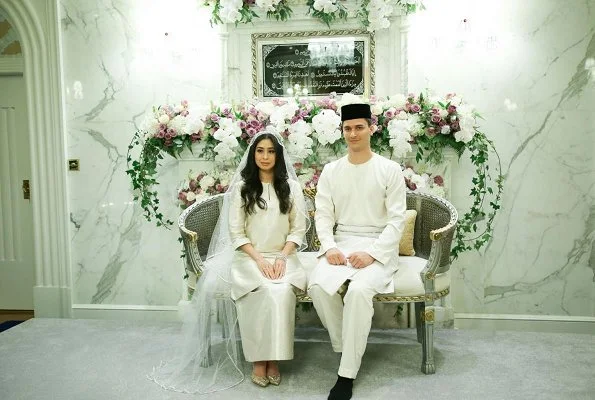The photograph, in landscape format, captures a couple on what appears to be their wedding day. They are seated together on a neatly arranged, gray couch that comfortably fits the both of them. The bride, distinguished by her long white veil pushed back from her face, sits beside the groom, who dons a black hat. Surrounding them is a lush array of maroon and white flowers intertwined with green vines, creating a breathtaking floral backdrop. Above them, a plaque with Arabic writing is prominently displayed on a highly reflective surface, adding a cultural touch to the scene. The room they occupy is splendidly adorned with marble from floor to ceiling, enhancing the elegance of the setting. To the right of the couple, part of an arched doorway is visible, further adding to the grandeur of the space.